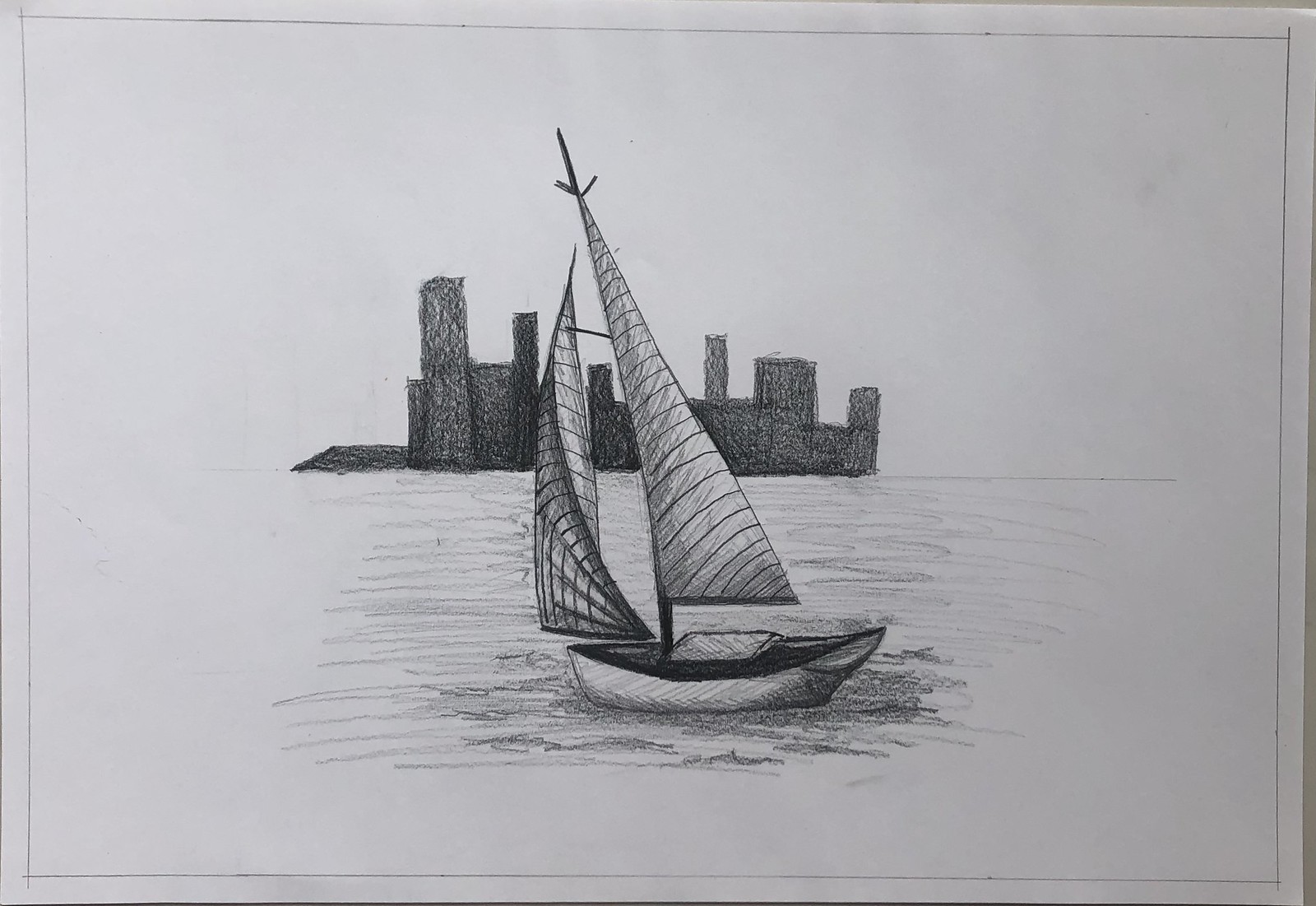This image is a photograph of an eight and a half by eleven-inch sketchbook page, turned sideways, featuring a detailed black and white pencil drawing. The artwork is framed by a very thin, lined border. The central scene showcases a small sailboat, approximately sixteen to eighteen feet in length, adrift on a calm sea. The boat, devoid of any visible crew, sports two sails with alternating light gray and black stripes; the front sail appears fully filled with wind, while the rear sail seems stiff and less affected by the breeze. The sailboat is slightly canted from right to left and tilted a bit toward the viewer, with noticeable shading indicating the sun's position—casting a darker shadow on the viewer’s side and underneath the boat.

The water is subtly rendered with pencil strokes, creating a simple, serene surface with minimal ripples. In the background, a cityscape emerges, comprised of blocky, solid black buildings of varying heights, suggesting the boat’s voyage towards an urban skyline. The sky above remains blank, free of any clouds or other details, emphasizing the stark contrast between the sea, the sailboat, and the silhouetted city beyond.